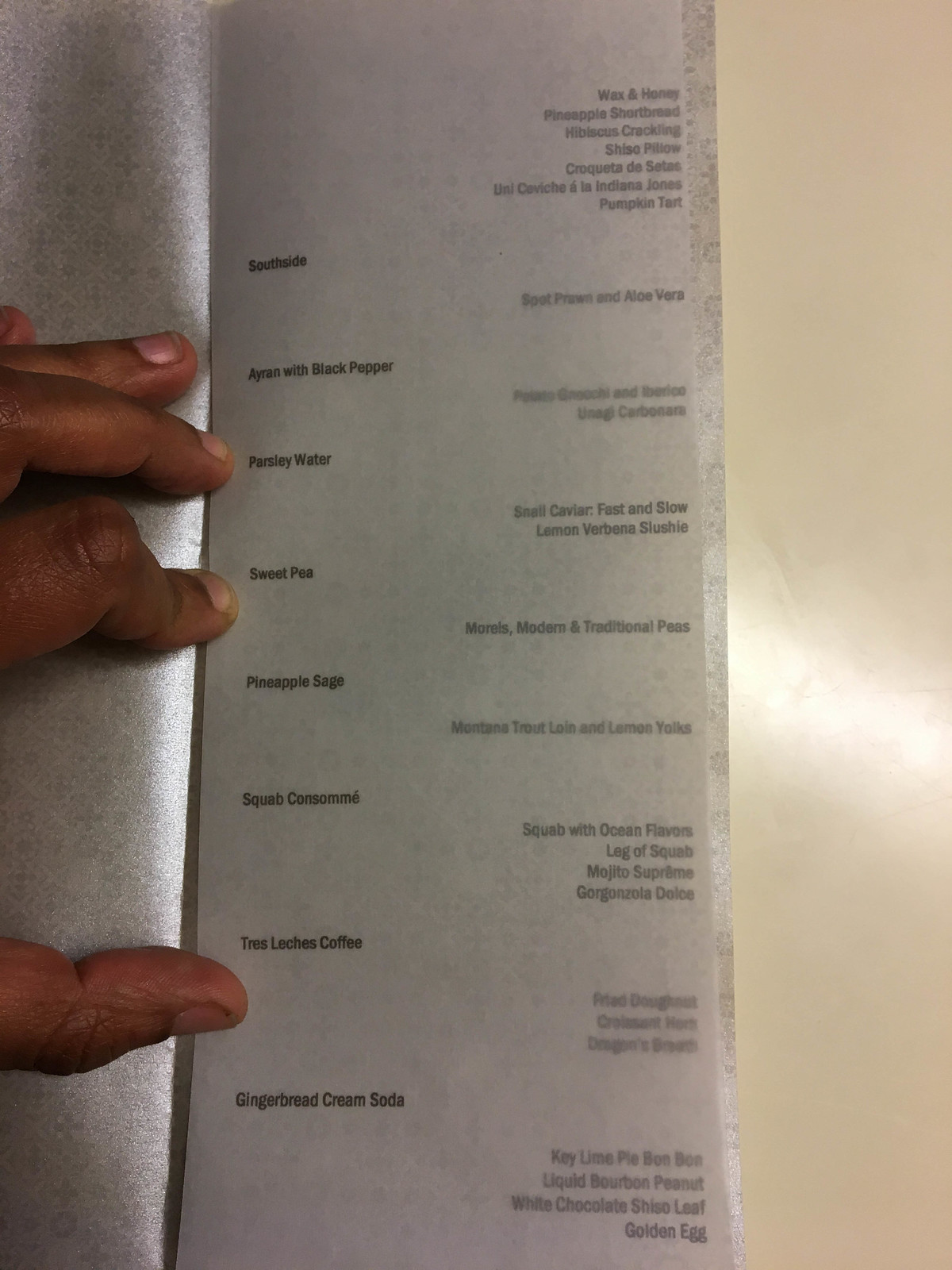A visually striking image of an elegantly designed menu being held open by an individual, showcasing an array of gourmet dishes. The menu is long and narrow, with a sophisticated silver cover that adds a touch of refinement. The dishes listed include unique and intriguing combinations such as beet, beets with aloe vera, caviar, fast and slow, lemon verbena slushy, morels, Montana trout, squash with ocean flavors, log of squash, and key lime pie. The hands of the person holding the menu frame the image, emphasizing their delicate grip and the silver cover that would otherwise obscure the detailed list of items. The overall color scheme of the photo is a soft blend of peach and light gray, creating a warm and inviting atmosphere.